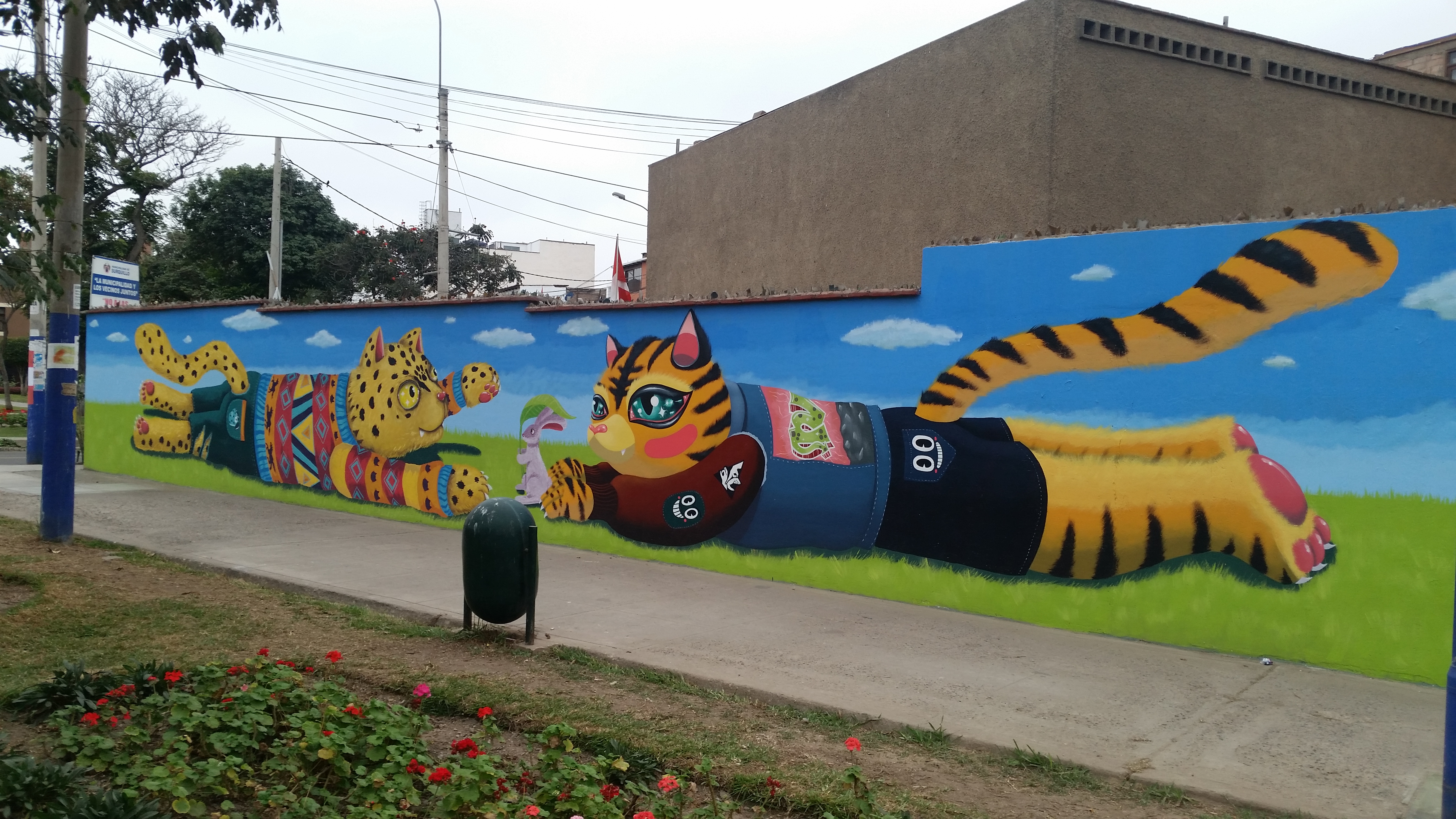This photograph captures an intricate and vivid mural along a concrete sidewalk in an urban outdoor setting, perhaps near a school or public building. Dominating the scene is a detailed mural painted on the side of a brown brick wall. The mural showcases two anthropomorphic cats with yellowish fur, one with tiger-like stripes and the other with leopard-like spots. These cartoonish cats are depicted lying on lush green grass under a blue sky dotted with white clouds. One cat is holding a pinkish rabbit, presenting it to the other, adding a playful and engaging element to the artwork. 

The mural is framed on the left by a garden area flourishing with green grass and vibrant red roses, contributing a touch of nature to the surroundings. In the background, one can see electrical poles and lines stretching into the white sky, as well as several trees scattered around, further emphasizing the urban landscape. The sidewalk itself is made of gray concrete and runs parallel to the mural, leading the eye along the vivid and colorful wall. Additionally, a round, cylindrical trash can stands nearby, subtly integrating everyday urban elements into this artistic scene.